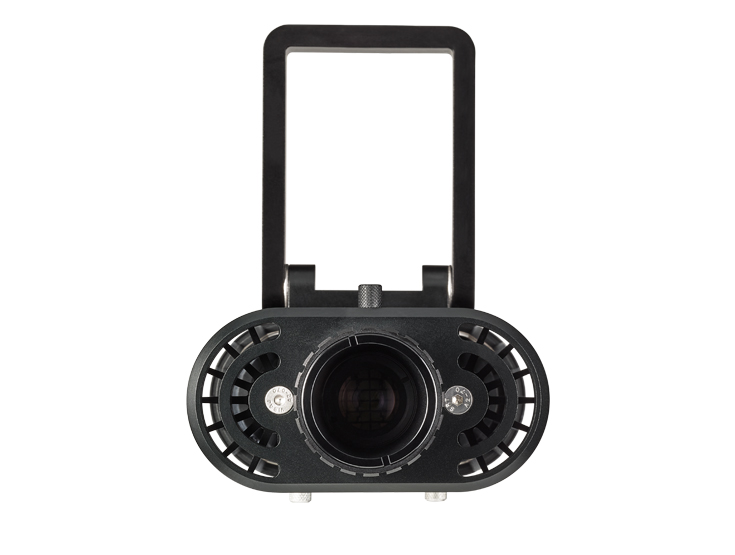The image features a sleek, black device that closely resembles a boombox or a music player, but it could also be perceived as a rudimentary camera or a projector. The central element is a prominent, circular black piece that looks like a lens, suggesting this area might function as a speaker magnet, camera lens, or projection point. Flanking this central lens-like structure are two silver screws or notes, adding a touch of metallic detail. The device has a very distinct, long black handle that arches over the top, providing easy portability. The background is a pure white, emphasizing the device's design. The overall form of the device is somewhat pill-shaped, being rounded on both sides, and it primarily features black and silver colors with precise silver linings accentuating its structure. There is no text in the image, and the perspective is a straight-on, frontal view, which makes it difficult to assess the depth and full functionality of the item.